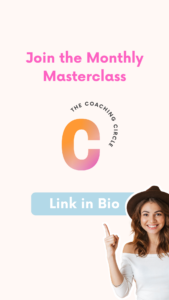The image is a vertically oriented advertisement, likely designed for display on a webpage accessible via computer or smartphone. The background is a flat, solid peachy-salmon color without any texture or gradient. 

Prominently featured in bubblegum pink text, positioned centrally and slightly down from the top, is the phrase "Join the Monthly Masterclass," with the letters "J," "M," and "M" capitalized. Just below this, there's a stylized "C" rendered in an ombre blend of orange, pink, and purple hues. Surrounding the "C," the arched text "the coaching circle" is displayed, echoing the curvature of the letter.

Towards the bottom part of the image, a blue banner with the text "Link in Bio" is shown in white. Adjacent to this, a girl with a black hat and an off-the-shoulder white shirt is pictured, pointing upwards towards the "Link in Bio" text.